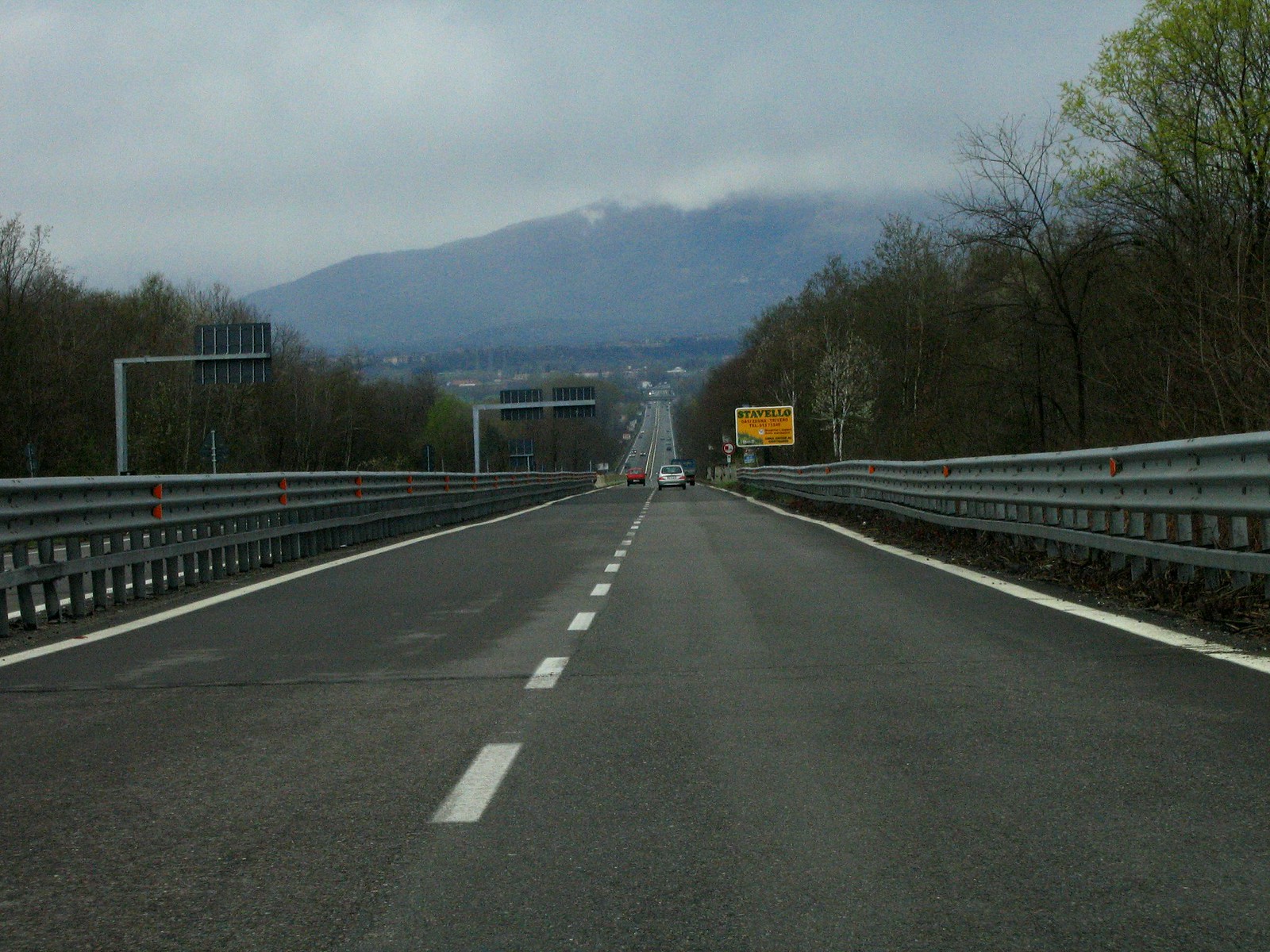This is a large square image captured from the right lane of a multi-lane freeway or highway. The scene is dominated by a cloudy sky, primarily gray with hints of white, giving the impression of impending rain. Toward the center of the picture, a faint outline of a hill or a foggy mountain is visible in the distance. The picture features a distinct view of the highway, with dotted white lines separating the lanes and solid white lines with guardrails on each side. There is a yellow sign with a white border in the middle of the image, possibly reading "Stavello." 

Several cars are seen traveling in both directions, primarily concentrated in the center of the image. Beyond the left guardrail, an adjacent road with street signs can be seen. The sides of the road are lined with trees, and there are indications of other structures like a couple of billboards and distant buildings. The color palette of the scene includes various shades of blue, white, gray, green, yellow, orange, red, and black. The environment appears to be outdoors, during the daytime, under overcast conditions. Red hazard lights are placed sporadically along the guardrails, contributing to the overall sense of caution and visibility on the foggy highway ahead.